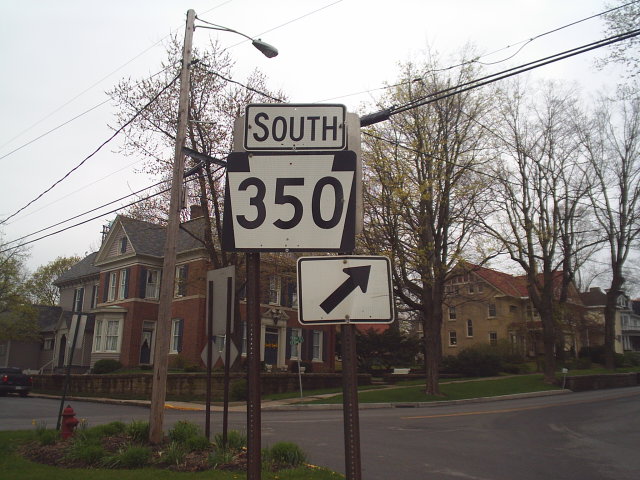This photograph captures a detailed street intersection scene dominated by a prominent road sign. The sign, a key focal point, features a bold black "South 350" inscription with the numbers "350" prominently displayed and a diagonal arrow beneath indicating direction. Surrounding this sign, a network of telephone and power wires crisscrosses the upper portion of the image.

In the foreground, to the bottom left, a red fire hydrant is nestled among green grass and shrubs. The intersection is bordered by a black-colored street and a well-kept sidewalk. Lining the sidewalk are large trees mostly bereft of leaves, hinting at a fall or winter setting.

In the background, the image reveals a series of four multi-level brick houses, including a Victorian-style, two-story home with several windows. Another building with brown brick and a red roof is also visible. Additionally, a red brick building with a black roof and white-painted windows can be seen across the street. The entire scene is under a gray, overcast sky, adding to the somber yet detailed ambiance of the photo.